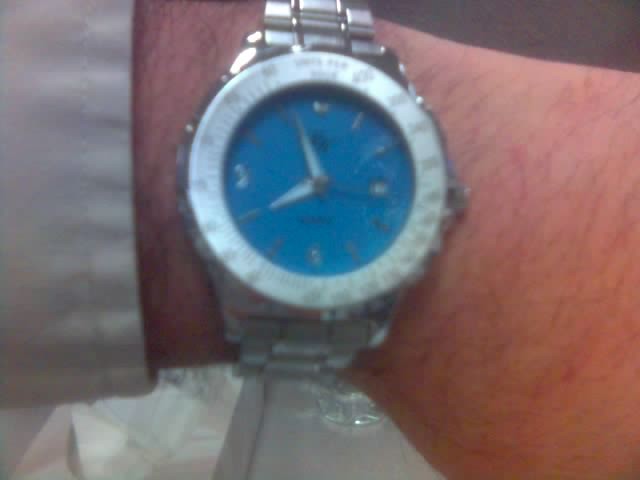This is a detailed photograph of a man's watch on a hairy wrist, which is coming in from the left side of the image. The wrist is adorned with a long-sleeved white dress shirt, featuring white stitching along the cuff, slightly visible towards the left. The man's wrist and hand, the latter extending to mid-hand, are tilted slightly downwards to the right, displaying black hair on the arm.

The watch is a large, round, silver men's watch with a silver metal wristband and a winding stem pointing to the right. The face of the watch has a silver border enclosing a medium blue face. The watch face displays silver numerals, with 12, 3, 6, and 9 depicted in a slightly different manner than standard numbers, creating a unique design. The remaining hour markers are represented by lines. Due to the way the light hits the watch, and a slight blur in the photo, some elements are not distinctly visible. The silver hands of the watch are positioned at either 7:55 or 7:59.

The background of the image transitions from a medium grey in the middle to a lighter, almost white grey at the left, with what appears to be a crumpled piece of cloth or paper. The upper right-hand corner of the background is darker, creating contrast with the lighter areas.